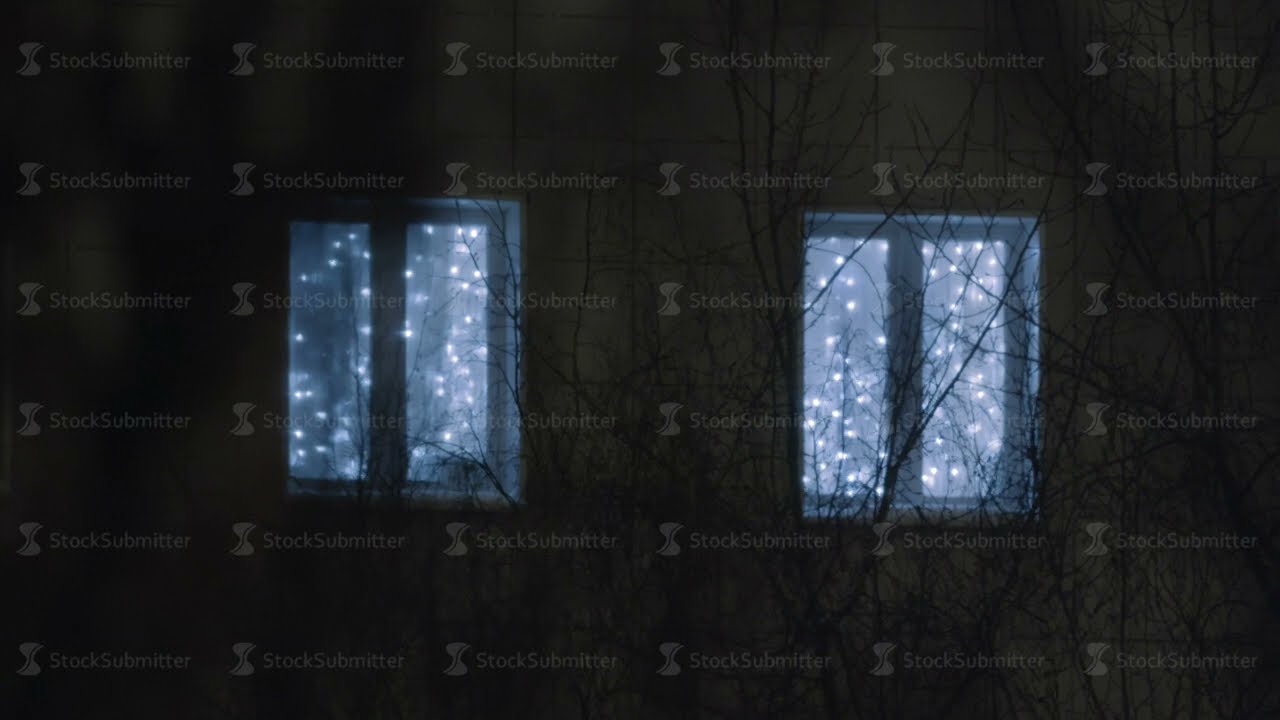The image depicts the side of a building taken at night, featuring two illuminated windows prominently centered in the photo. Each window is divided by thin vertical panes, resulting in a total of four window panes visible. Behind the windows is white fabric and small, twinkling fairy lights, which resemble tiny stars scattered across the backdrop. Outside, bare tree branches, devoid of leaves and sharply silhouetted against the lighted windows, intersect the scene, adding a stark contrast against the brightness within. The entire image is overlaid with a repetitive watermark that reads "stock submitter," accompanied by an hourglass or figure-eight shape to the left of the text. This watermark is uniformly distributed in a grid pattern across the photograph. The overall ambiance of the image is dark, emphasizing the glowing warmth spilling out from the windows, with no other objects or text visible aside from the mentioned watermark.